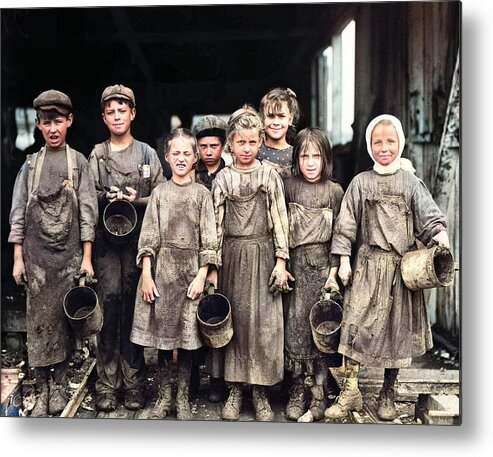The image is a square photograph capturing a group of eight children standing in front of a dilapidated wooden structure, possibly an old warehouse or factory. The group is a mix of five girls and three boys, all of whom look very young, most likely children or early teenagers. They appear impoverished and are dressed in worn, dirty clothes covered in a grayish, soot-like grime. The boys on the left wear shirts, pants, and aprons, with popper-style hats perched on their heads. The girls on the right are clad in long-sleeve dresses, also with aprons. Interestingly, one girl positioned in the center left wears only a dress without an apron. All of the children are holding large canisters with handles, suggesting that they might be carrying water. Despite the grimy and disheveled appearance that gives them a much older look, some of the children are smiling while others have more somber expressions. Their light-colored skin and hair stand out amidst the otherwise black-and-white, almost monochromatic scene. They all wear boots, indicating that they might have just finished or are in the midst of doing laborious work.